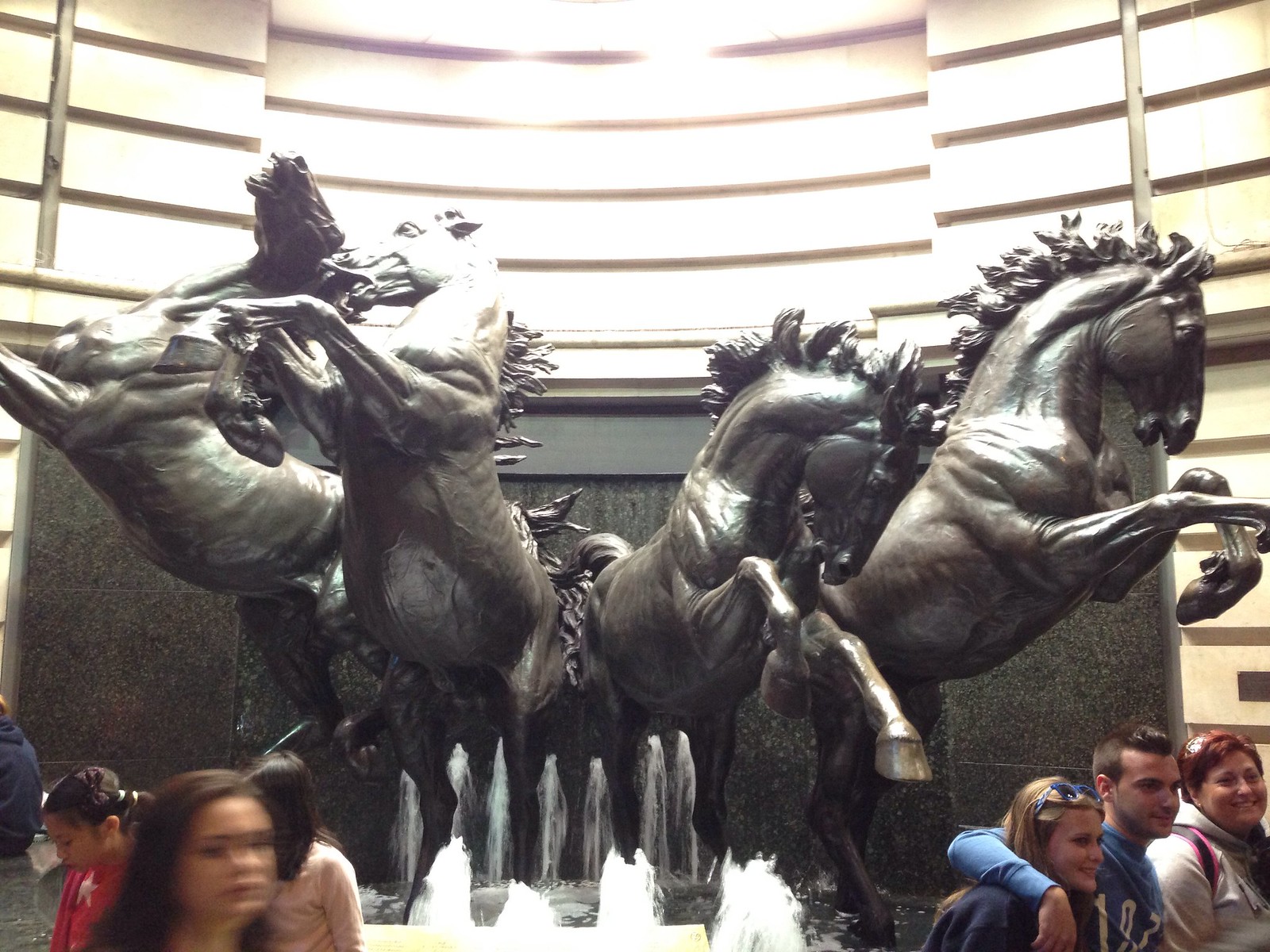The image depicts a detailed and dynamic sculpture arrangement of four black horse statues inside what appears to be a museum. Each horse is rearing up on its hind legs with their front hooves raised, exuding a sense of motion as their manes appear windswept. The two horses on the left are angled towards the left, and the two on the right are angled to the right. Beneath the horses, there is a flowing fountain, water cascading around the statues and adding a sense of grandeur to the scene. The backdrop features a majestic white, curved, and beveled wall illuminated by overhead lights, enhancing the ethereal atmosphere. Surrounding the fountain, numerous visitors can be seen, some blurred due to motion, immersed in taking photos and engaging with the exhibit. Notable among the onlookers are a woman in a red shirt and another in gray, capturing the diversity of attire among the observers. The intricate detail of the horse statues, with visible texturing of their skin and hair, adds to the lifelike illusion, making the scene both visually striking and lively.